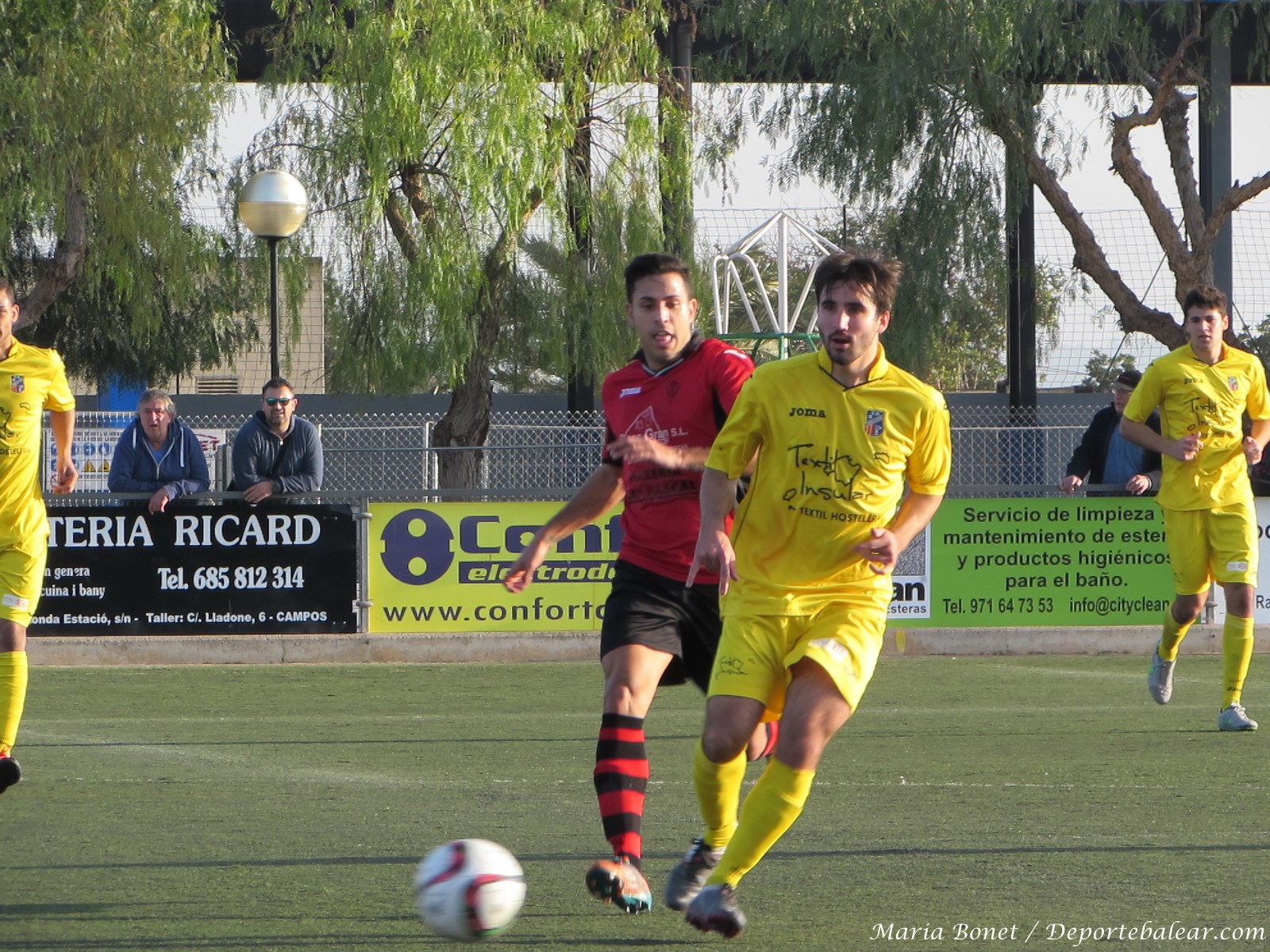This image captures an outdoor European football match on a large grassy field marked with white lines. Central to the photograph, several soccer players are intensely chasing a ball. The players are decked out in distinct uniforms: some in yellow shirts, shorts, and socks, and one player in a red shirt with black shorts and black-and-red striped socks. Surrounding the field, there are various details including fences, buildings, light poles, and trees. Spectators can be seen leaning over the fences; two are on the left-hand side, and one is on the right-hand side of the image. Advertisements along the fence include a telephone number (685-812-314) and text such as "Servicio de Limpiza Maintenimiento de Estereoproductos Higienico para el Bano." The bottom right corner of the image includes a watermark reading "mariebonnettdeportballier.com." The photograph seems to be taken in broad daylight, with vibrant colors including green, white, red, black, yellow, silver, gray, and blue, all contributing to the lively atmosphere of the game.